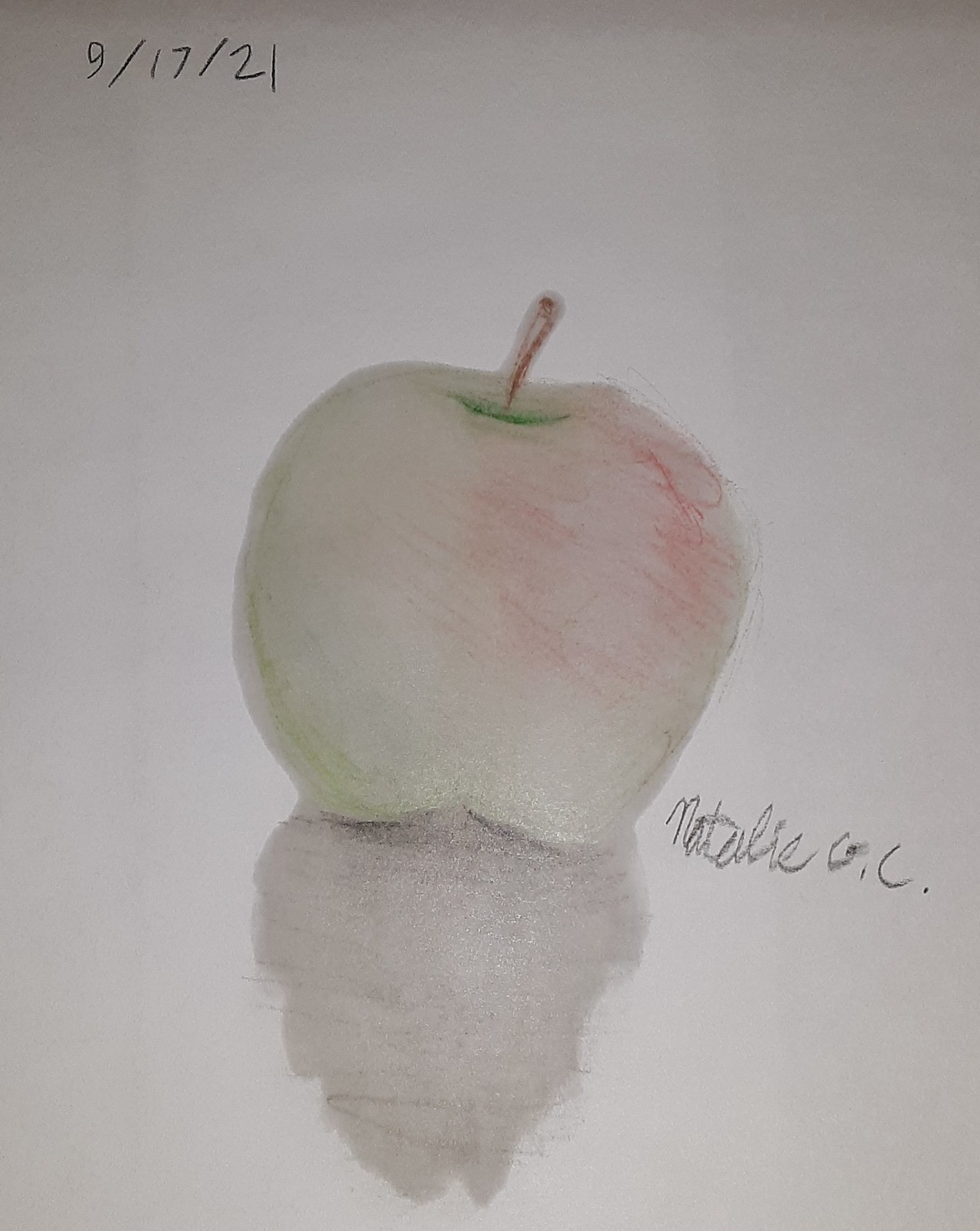This image showcases a detailed sketch of an apple, set against a light grey background. The apple, which appears deformed, features a brown stem and a complex array of colors: a green lining inside, a pale red shading on the right, and mixed shades of off-white, red, and green in the middle. The apple is slightly tilted to the right, casting a darker, distorted shadow beneath it that is more angular and irregular in shape. In the upper left corner, the date "9-17-21" is inscribed. On the right side of the apple, the black signature reads "Natalie C.C.," likely the artist. The overall image is a nuanced and color-rich representation that combines traditional sketching techniques with an abstract twist.